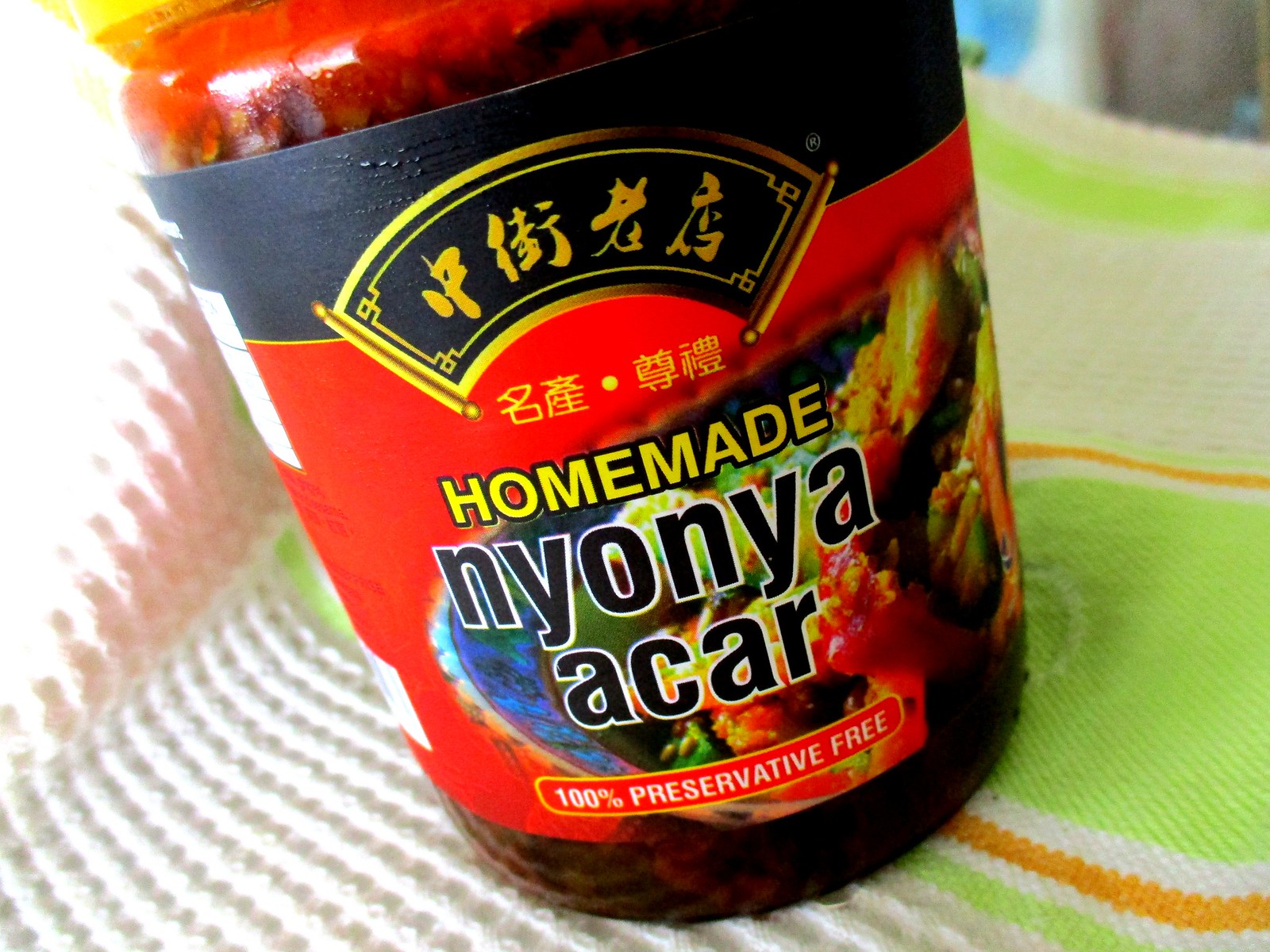This close-up image features a medium-sized transparent jar of Homemade Nyonya Acar, titled in English with a subtitle declaring it 100% Preservative Free. Above the title, there is a logo in black and gold and some text in Mandarin. The jar is filled with a dark red condiment that resembles a chili-colored sauce, possibly with bits of cooked cucumber visible through the glass. The jar has a yellow lid. The label is red and shows an example of the food in a bowl. The jar is placed on a white kitchen towel, which has green and orange sections, against a slightly blurry background.